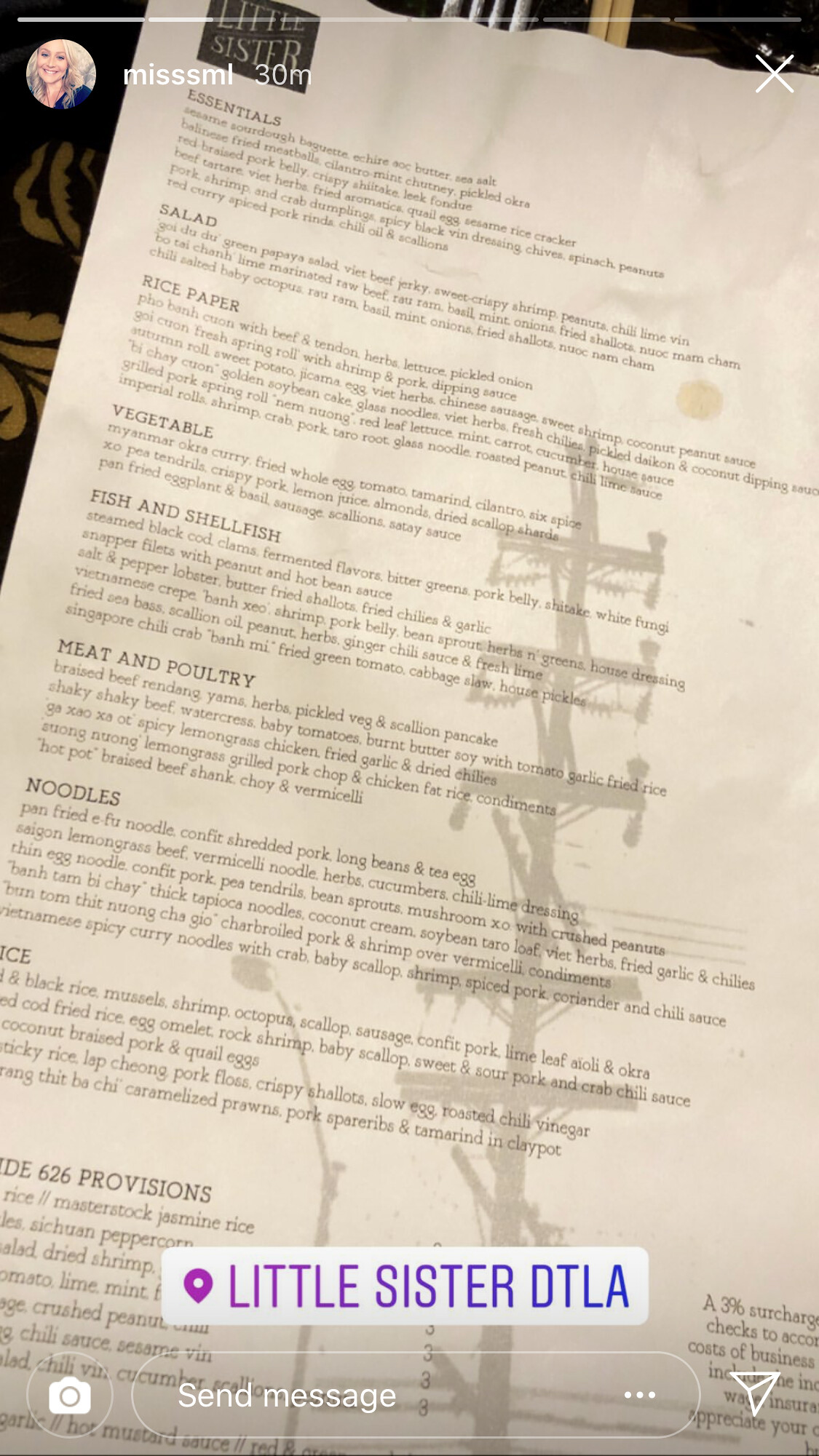The image is a detailed screenshot of an Instagram story. In the top left corner, there's a profile photo bubble of a blonde woman. Next to this, the narration indicates that the caption's author is a young man. The photo prominently features a menu titled "Essentials."

At the top left, there is a black square labeled "Little Sister." The center of the image displays what appears to be an electric pole or tower. There is also a lamppost situated towards the bottom left. Adjacent to it, there's another square, and a circle can be seen at the top right of the image.

The left side of the menu lists various food sections and items including: 
- Sesame Sourdough Baguette
- Butter, Sea Salt
- Fried Meatball with Cilantro, Mint Chutney, and Pickled Okra
- Red Rice, Purple Lettuce, Crispy Shiitake, Leek, Fondue
- Beef Tartare with Herbs
- Fried Eggs, Cold Eggs
- Sesame Rice Cracker
- Pork, Shrimp, and Crab Dumplings
- Spicy Black Bean Dressing
- Fried Spinach
- Peanuts, Fried Curry, Fried Pork Rind
- Chili Oil
- Scallions
- Salad, Rice Paper
- Various selections under Vegetables, Fish and Shellfish, Meat and Poultry, and Noodles.

At the very bottom of the menu, it states "Little Sister, DTLA" in a white rectangle with purple text, indicating the location of the establishment. Additionally, the bottom left features a camera icon, and the bottom section contains phrases like "send message" with three ellipses and an arrow pointing to the right.

The bottom right of the image notes a policy about costs of business, ending with an incomplete phrase: "Represent search hard text to account cost of business including something appreciated or something." 

While the menu is extensive, the caption suggests that reading all the items would be too extensive for this description.